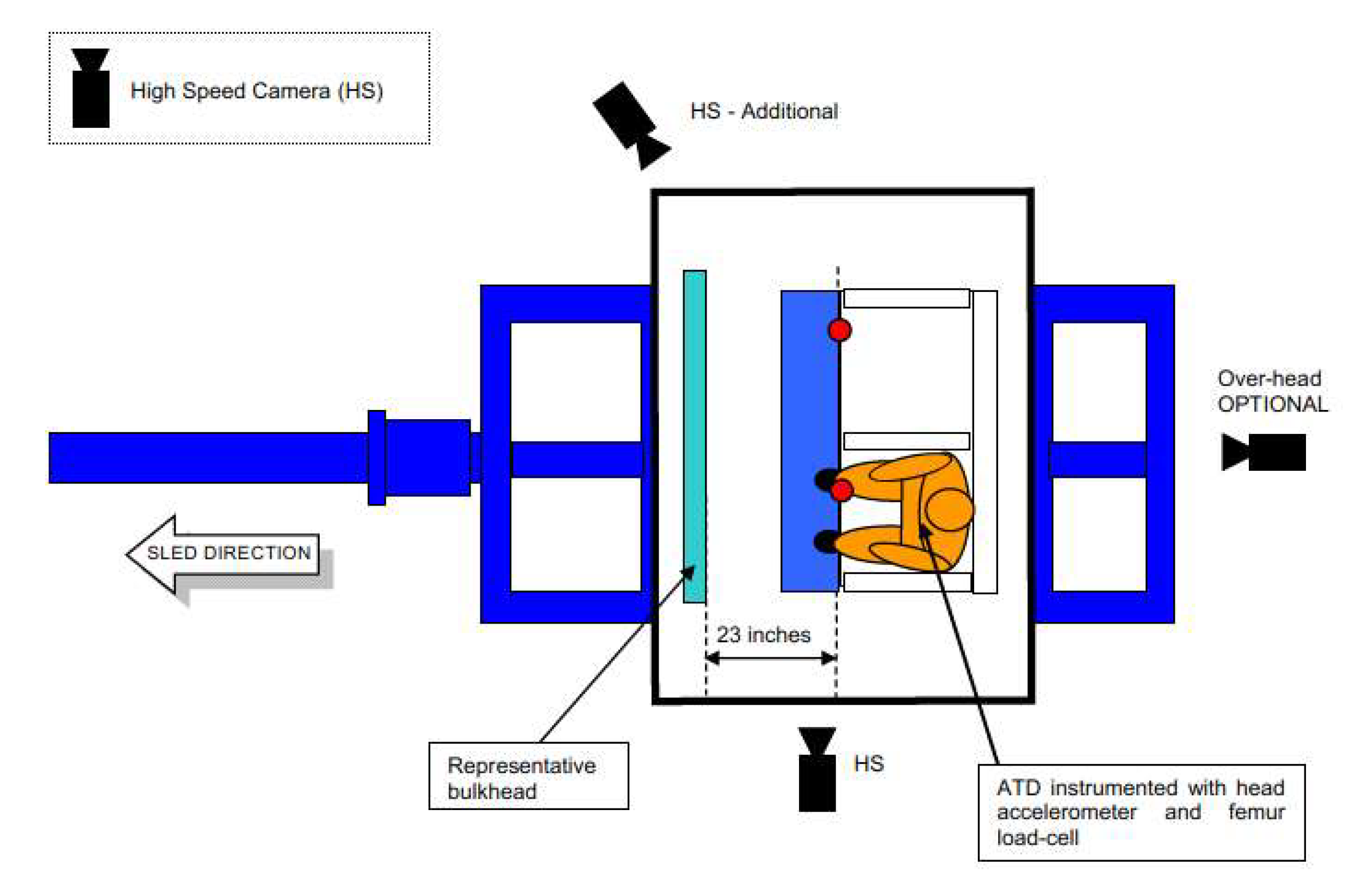The hand-drawn aerial diagram illustrates a detailed setup involving a human figure and various pieces of equipment, all contained within a black-outlined vertical rectangle. The orange human figure, outlined in black, is seated on the left side of a two-seat configuration, with the adjacent seat empty. Directly in front of the figure is a green line labeled "Representative Bulkhead," indicating a 23-inch spacing from the figure's feet to the bulkhead. The person is marked as "ATD Instrumented with Head Accelerometer and Femur Load Cell," suggesting the presence of specific measurement devices.

The diagram features several blue double-pane window-like areas on both the left and right sides, with the left blue pane connected to a pipe-like structure. Beneath this structure, a white arrow labeled "SLED Direction" points to the left.

Three black solid images of cameras are strategically placed around the rectangle, aimed at the seated figure. The camera at the top left is labeled "HS Additional," the one to the right of the blue right rectangle is labeled "Overhead Optional," and the bottom camera is labeled "HS."

In the upper left-hand corner, there is a notation, "High-Speed Camera (HS)," emphasizing the nature of the cameras involved in this setup. The entire scene is colored with a mix of royal blue for framework, orange for the human figure, green for the bulkhead, and teal for the representative bulkhead bar, creating a clear yet intricate visual depiction of the testing or observational setup.